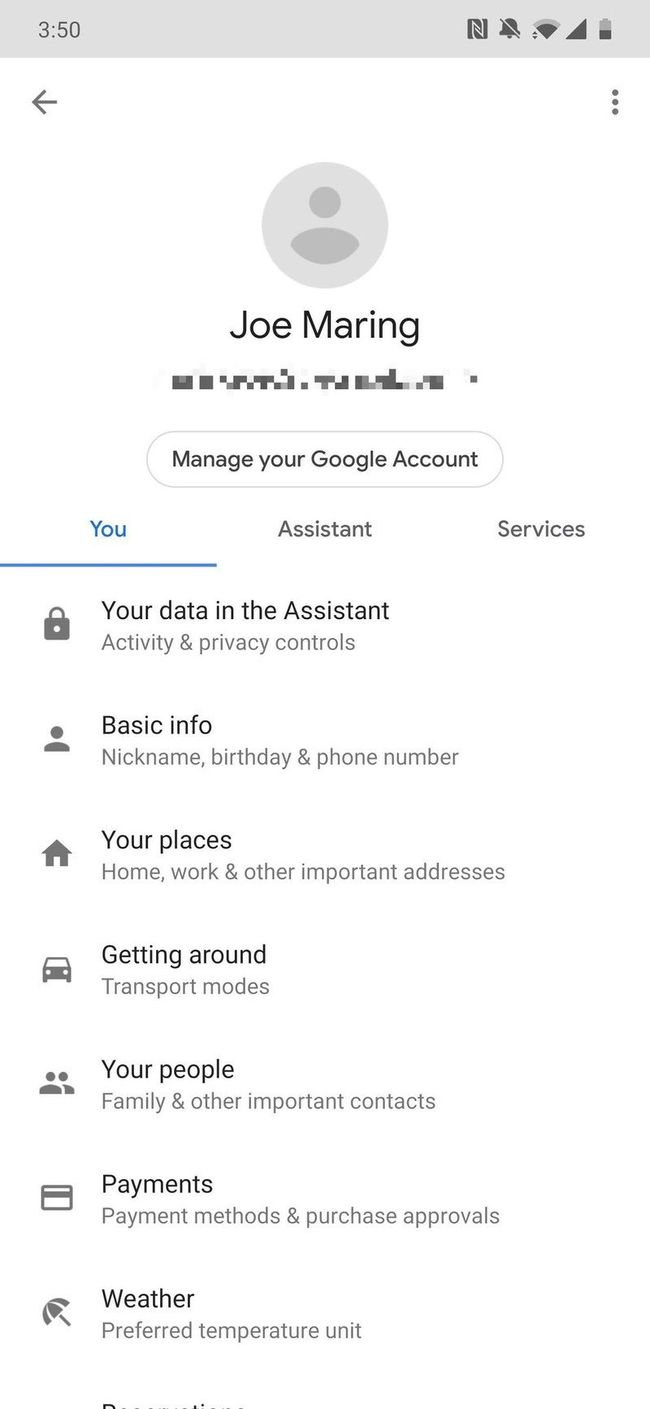This is a detailed screenshot of a Google account page displayed on a mobile device. At the top of the screen, the user's name, "Joe Mooring," is prominently shown. Above the name, there is a default user avatar icon. Beneath the name, however blurred for privacy, is a contact information section. Just below this section, there is an option to "Manage your Google Account" accompanied by a round button. 

Further down, three tabs are visible: "You," "Assistant," and "Services." The "You" tab is highlighted in blue with a blue underline, indicating it is currently active. This section contains a list of seven items, each marked with distinct icons to the left and descriptive text to the right. The items listed include "Your data in the Assistant," "Basic info," "Your places," "Getting around," "Your people," "Payments," and "Weather."